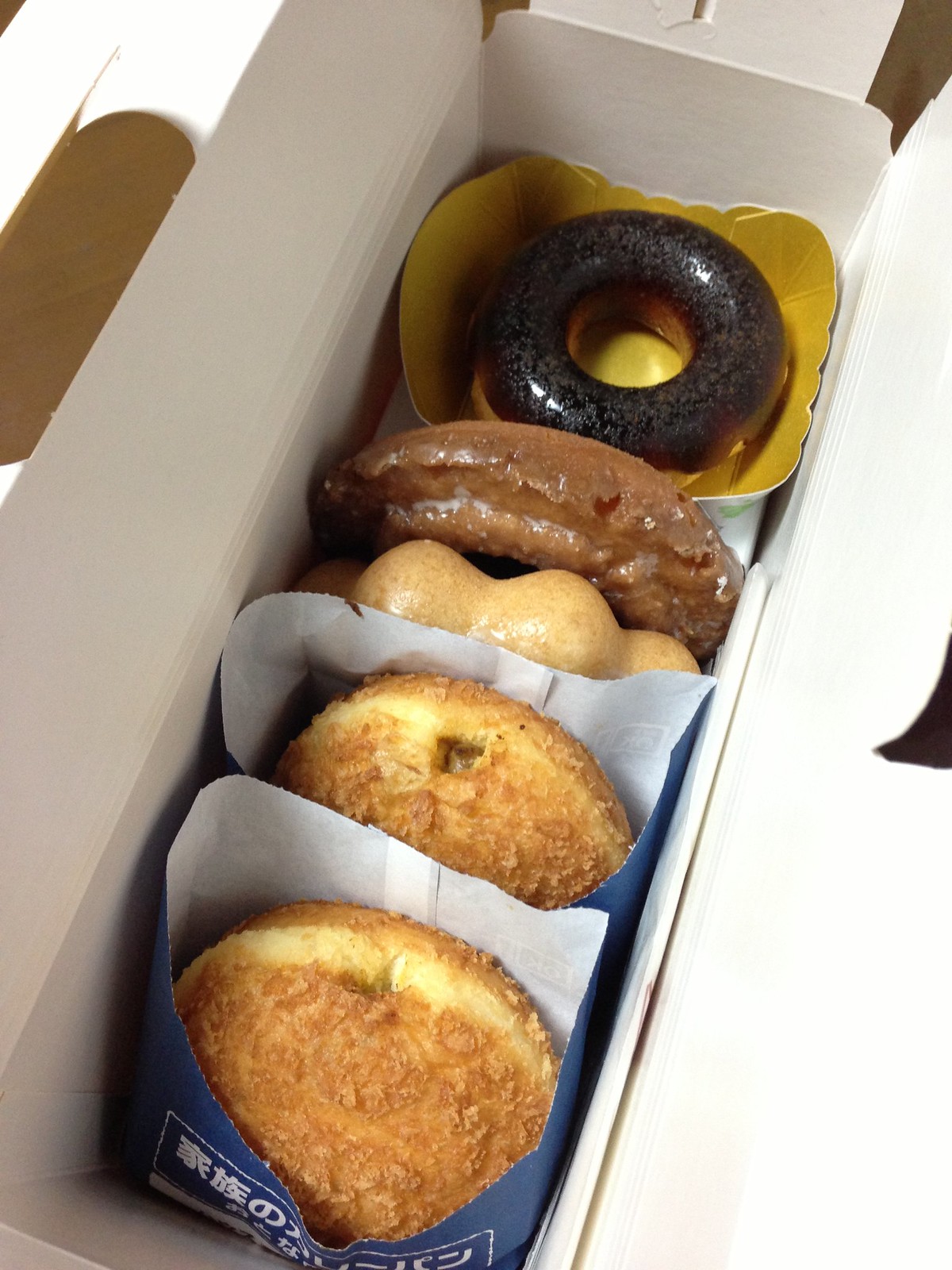This photograph depicts a white rectangular box containing five assorted donuts. In the upper section, there's a chocolate-topped cake donut nestled in a yellow plastic container, next to an old-fashioned glazed donut with a distinctive, crispy surface. Nearby is a French cruller with curved, flower-like edges. The bottom section houses two donuts in blue paper sleeves marked with Chinese characters, indicating they might be from a small, locally-owned or culturally diverse bakery. Each of these two donuts appears to be filled, possibly with jelly, given the small holes in their centers. All the donuts, varying in textures and delightful glazes, suggest a rich assortment from a unique bakery.